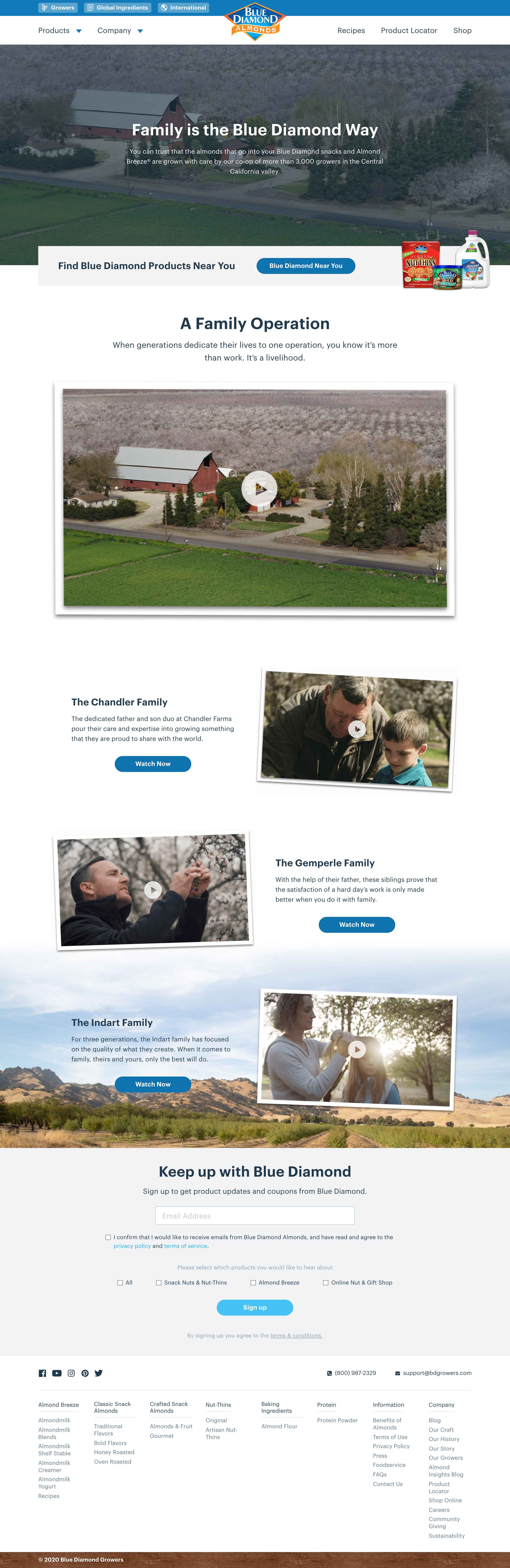The image features a webpage with a layout that's somewhat unclear due to its blurriness. At the top, there is a prominent blue bar centered with the Blue Diamond logo. Below this, there's a picture with a grayish tint, depicting a farmhouse, a field, and some trees. Overlaid on this image is the phrase "Our family is the Blue Diamond way," with some text underneath that is difficult to read. Further down the page, there is a noticeable blue button whose function isn't specified, situated next to a container, possibly a box.

In the section labeled "The Family Operation," another image of a farmhouse and field is displayed, this time with a play button in the center, indicating it is a video. To the left of this video, there's a paragraph, and to the right, a picture of two individuals. Below this, another section mirrors the layout, with a picture on the left of one person and a paragraph on the right. Continuing further down, there's one more paragraph positioned to the left and a picture of someone on the right.

At the bottom of the webpage, the text "Keep up with Blue Diamond" appears above a box where users can presumably enter their email address to stay updated.